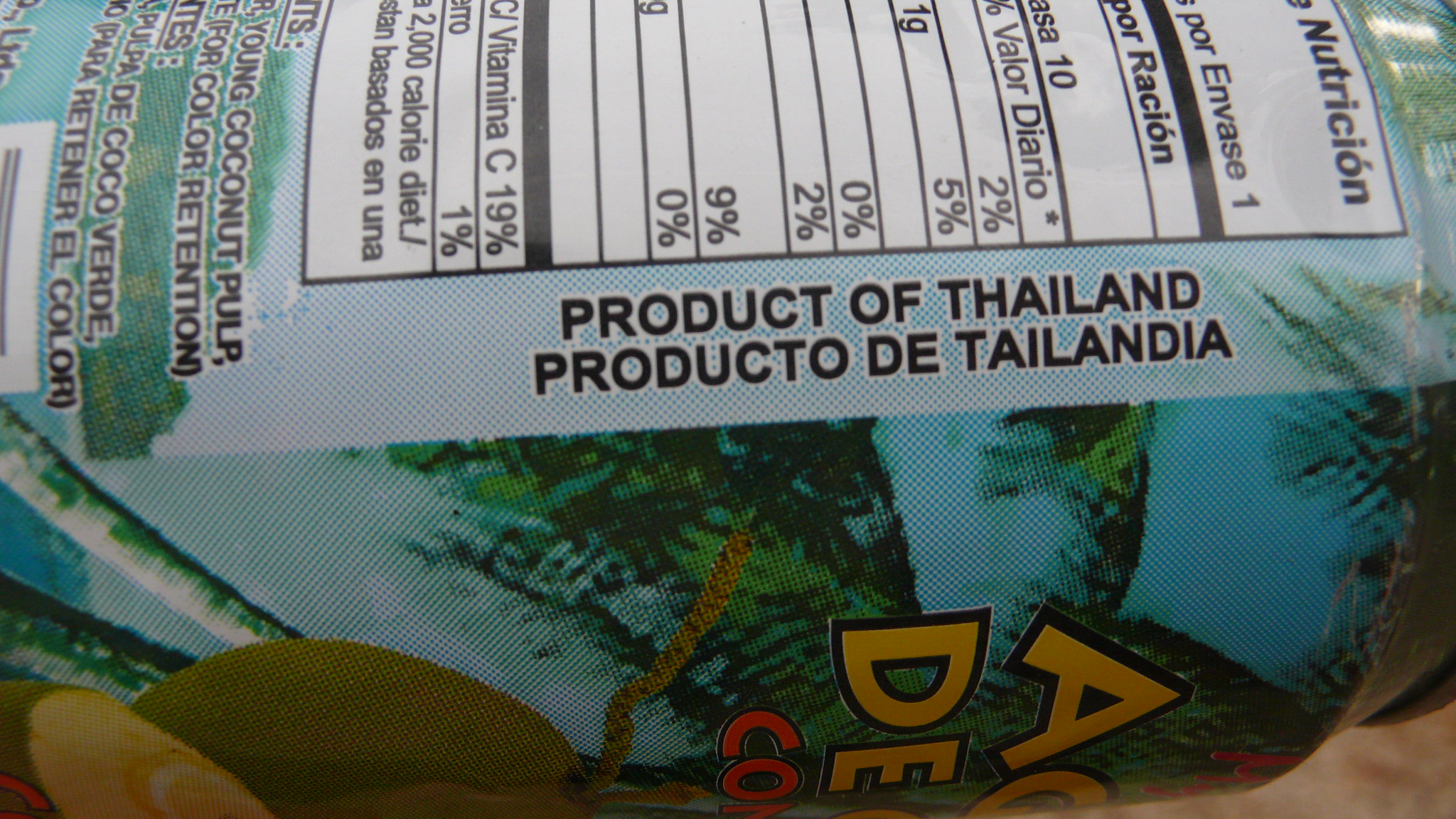This image showcases the side profile of a horizontally positioned can, prominently featuring an eclectic beach scene complete with coconuts and swaying palm trees set against a serene backdrop. The can's design displays a mix of text orientations; some text appears upright, while other parts are presented sideways due to the can's orientation. In striking black text, the can reads "Product of Thailand" followed by its Spanish equivalent, "Producto de Thailandia." Positioned above this text is a neatly organized white and black rectangle containing nutritional facts, vital for any discerning consumer. Below this nutritional information is a section featuring a list of ingredients in dark black text, alongside a slight glimpse of a barcode at the edge. Towards the bottom of the can, vibrant yellow and orange fonts announce the name of the beverage, adding a pop of color and attracting attention to the product's branding.